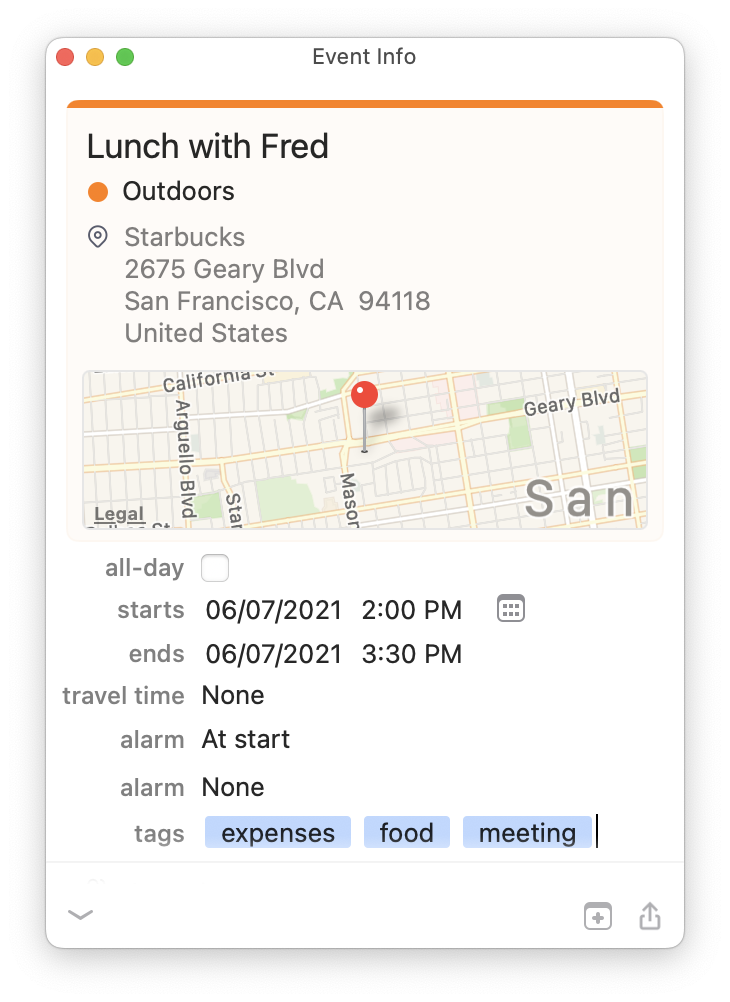The image is a detailed screenshot of a calendar event interface, predominantly white with orange accents. At the top of the interface are three circular buttons in red, orange, and green. Centrally positioned is the heading "Event Info."

An orange bar spans the width of the screen, prominently displaying "Lunch with Fred" in bold black text. Adjacent to this is an orange dot with the label "outdoors," indicating the location as Starbucks at 2675 Geary Boulevard, San Francisco, California, 94118. A small map pin highlights the intersection of Geary Boulevard and Mason.

Below, there is an unchecked box labeled "All day." The specifics of the event show it starts on June 7th, 2021, at 2:00 p.m. and concludes at 3:30 p.m., with no allocated travel time. The alarm is set to go off at the start of the event. The tags associated with this event are "expenses," "food," and "meeting," highlighted in blue.